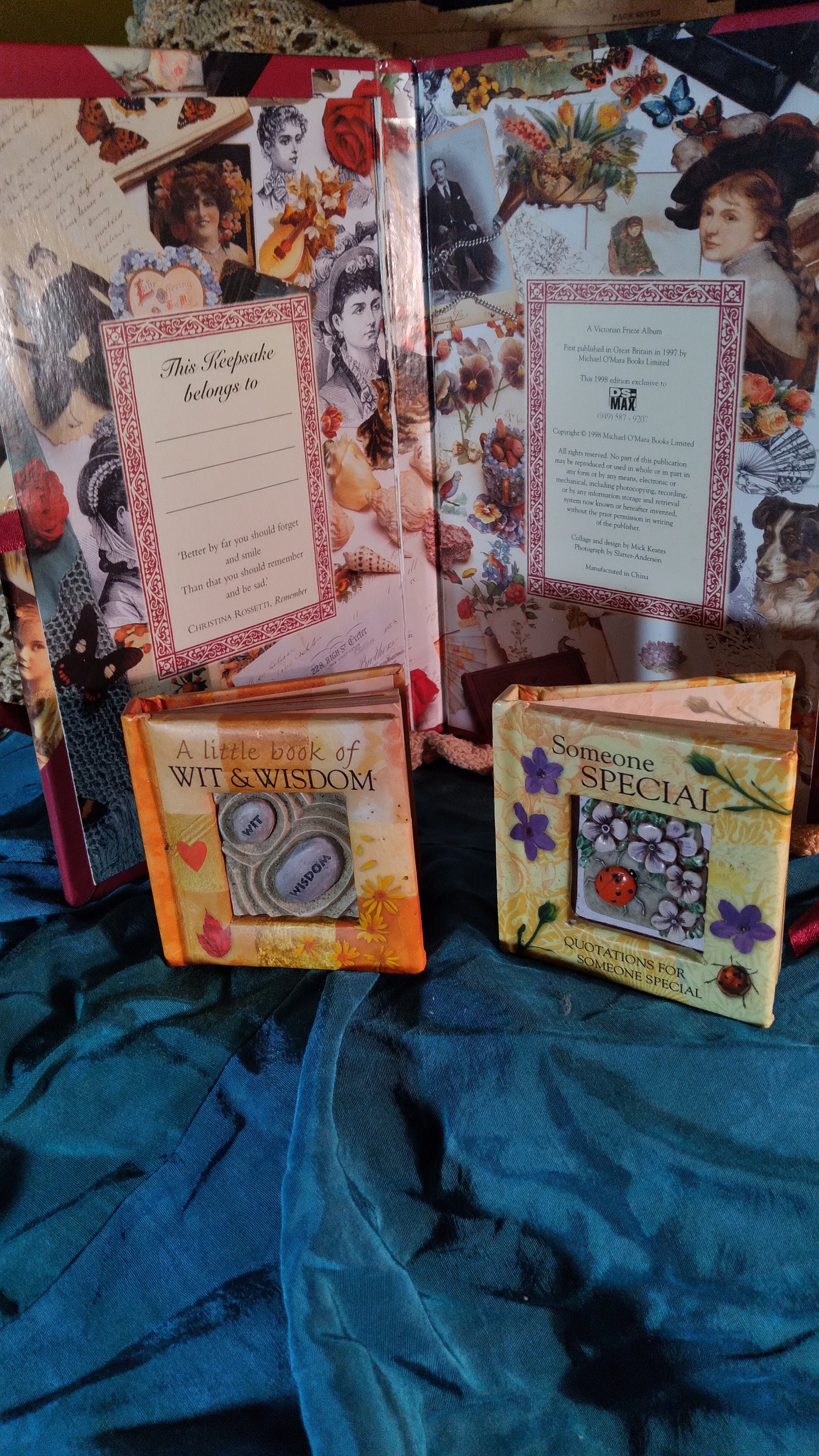In this indoor photograph, several books are artfully arranged on a blue cloth. The main book, which is open to a two-page spread, features various portraits of people on the left-hand page. The right-hand page includes the text "This keepsake belongs to" followed by lines for personal inscriptions. Below it, a quote from Christina Rossetti reads: "Better by far you should forget and smile than you should remember and be sad." There is another block of text on this page, but it is partially obscured.

In front of the main book are two smaller volumes. The closest one is titled "A Little Book of Wit and Wisdom," adorned with an illustration resembling a sand garden, complete with two stones labeled "Wit" and "Wisdom." To its right lies another book titled "Someone Special," featuring a charming pattern of ladybugs and flowers with the subtitle "Quotations for Someone Special." The overall presentation on the blue cloth creates a cozy and thoughtful ambiance, emphasizing the themes of memory, wisdom, and special connections.